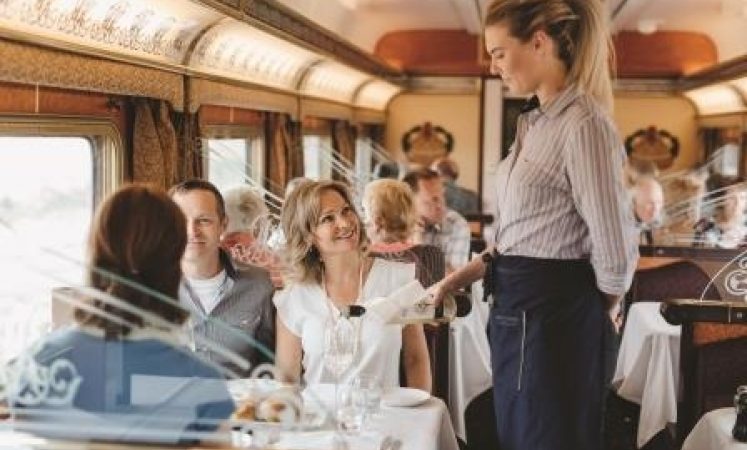This image captures the luxurious dining car of a train, brimming with elegance and attention to detail. The spacious interior is adorned with rows of seating booths on either side, each designed to accommodate four diners with comfort and style. Each table is covered with a pristine white tablecloth, creating a refined dining atmosphere. On the left side, a blonde woman with shoulder-length hair, dressed in a white top and necklace, is seated next to a man, likely her partner. She is looking up and smiling at a waitress who stands in the central aisle, serving their table. The waitress has sandy blonde hair pulled back in a ponytail and is wearing a long-sleeved collared dress shirt with light brown vertical stripes, complemented by a dark-colored apron around her waist. She is pouring white wine into the glass of another female diner seated across from the couple. The dining car boasts wooden seating booths, further enhancing the luxurious feel. The other tables are occupied by passengers, separated by glass partitions atop the seatbacks, adding both privacy and elegance to the scene.